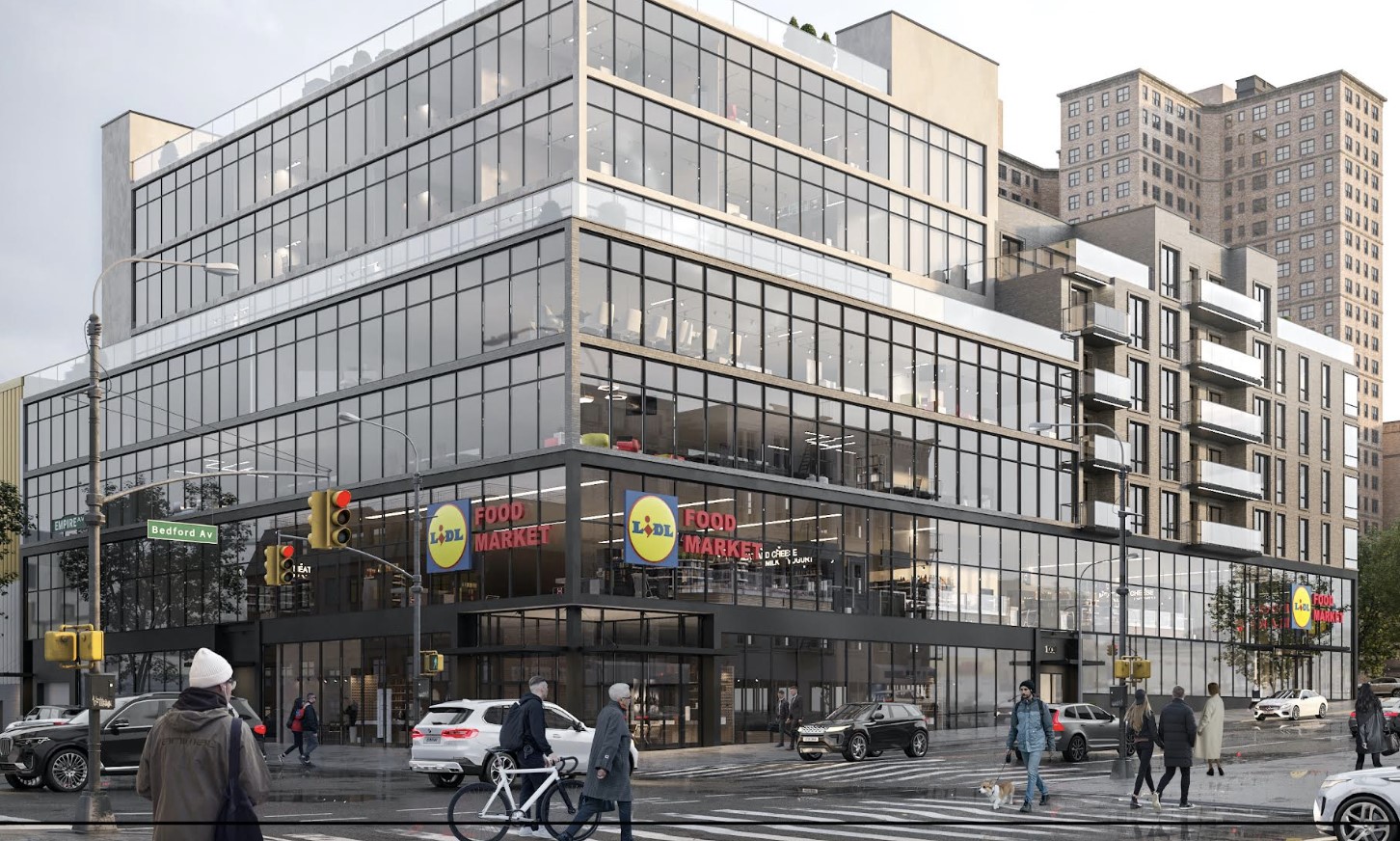In this image, a bustling downtown area is prominently featured. Central to the scene is a large six or seven-story building with an exterior completely lined with numerous windows, providing a modern and sleek architectural look. At the very top of the building, there is a rooftop garden area, adding a touch of greenery amidst the urban landscape. 

The ground level houses a store identified by its signage as "LIDL Food Market," which seems to occupy the first two stories of the building. The upper stories, with their many visible windows, reveal office-like spaces complete with cubicles and chairs, suggesting that the floors above the market are used as office spaces.

In the background, attached to the primary structure, are apartment-style buildings, blending residential spaces into the urban framework. The scene also captures a red traffic light, with a street sign indicating the intersection of Bedford Ave and Empire Ave.

The atmosphere is somewhat gloomy, indicative of either a rainy day or generally overcast weather. The streets are alive with activity; numerous pedestrians are seen walking, including a man with a dog. There are also several cars in motion and a white bicycle in view, painting a picture of a vibrant and busy city life.